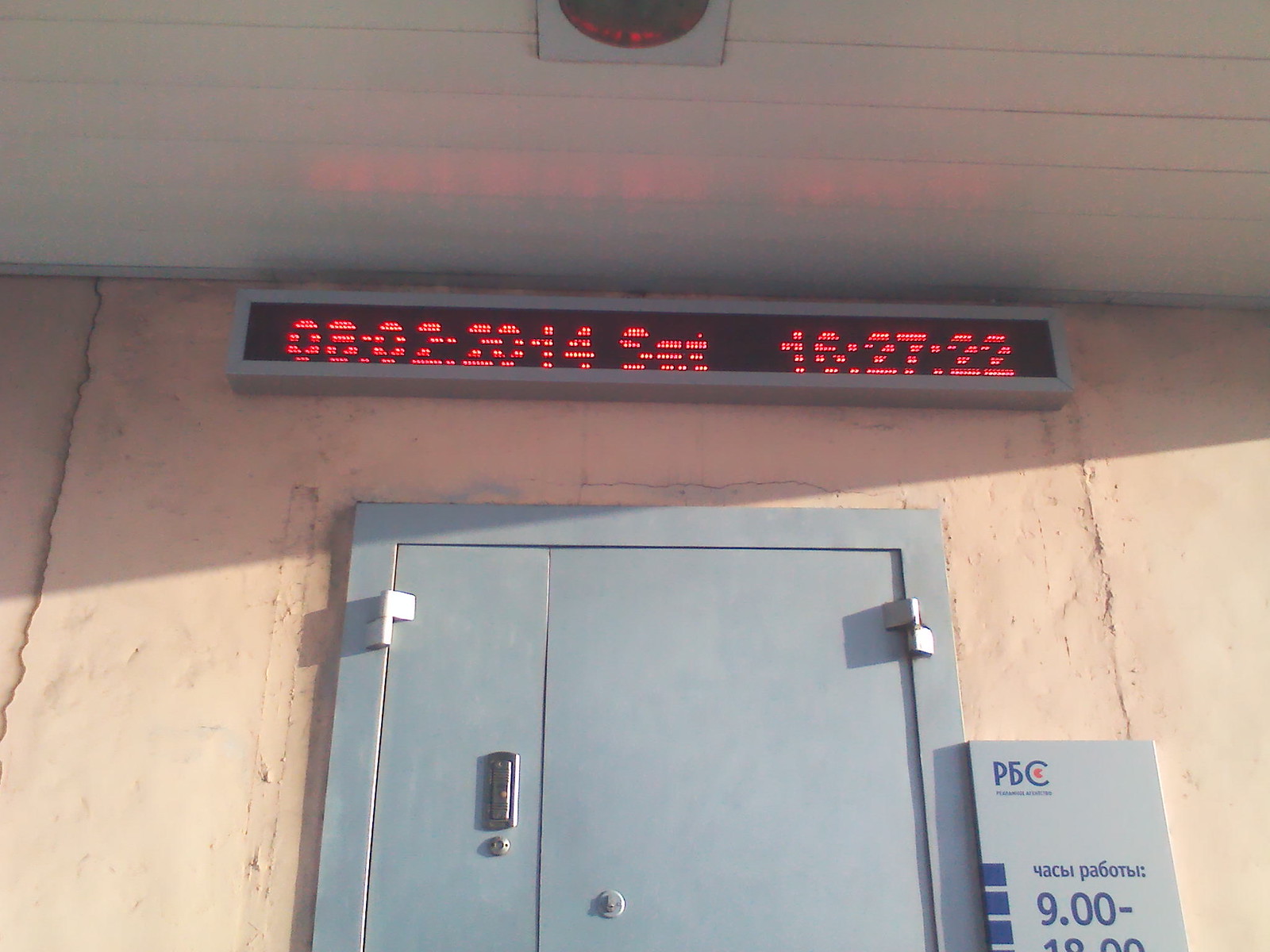An outdoor movie theater with a distinctly European ambiance, possibly located in a Czech-speaking region, judging by the text on its signage. The marquee, featuring standard movie theater times, stands prominently. The structure includes weathered blue doors and a similarly colored sign, set against a backdrop of deteriorating walls that hint at the venue's age. Despite its somewhat worn appearance, the setting maintains a certain charm and functionality, blending the nostalgia of classic cinemas with the unique experience of outdoor viewing.